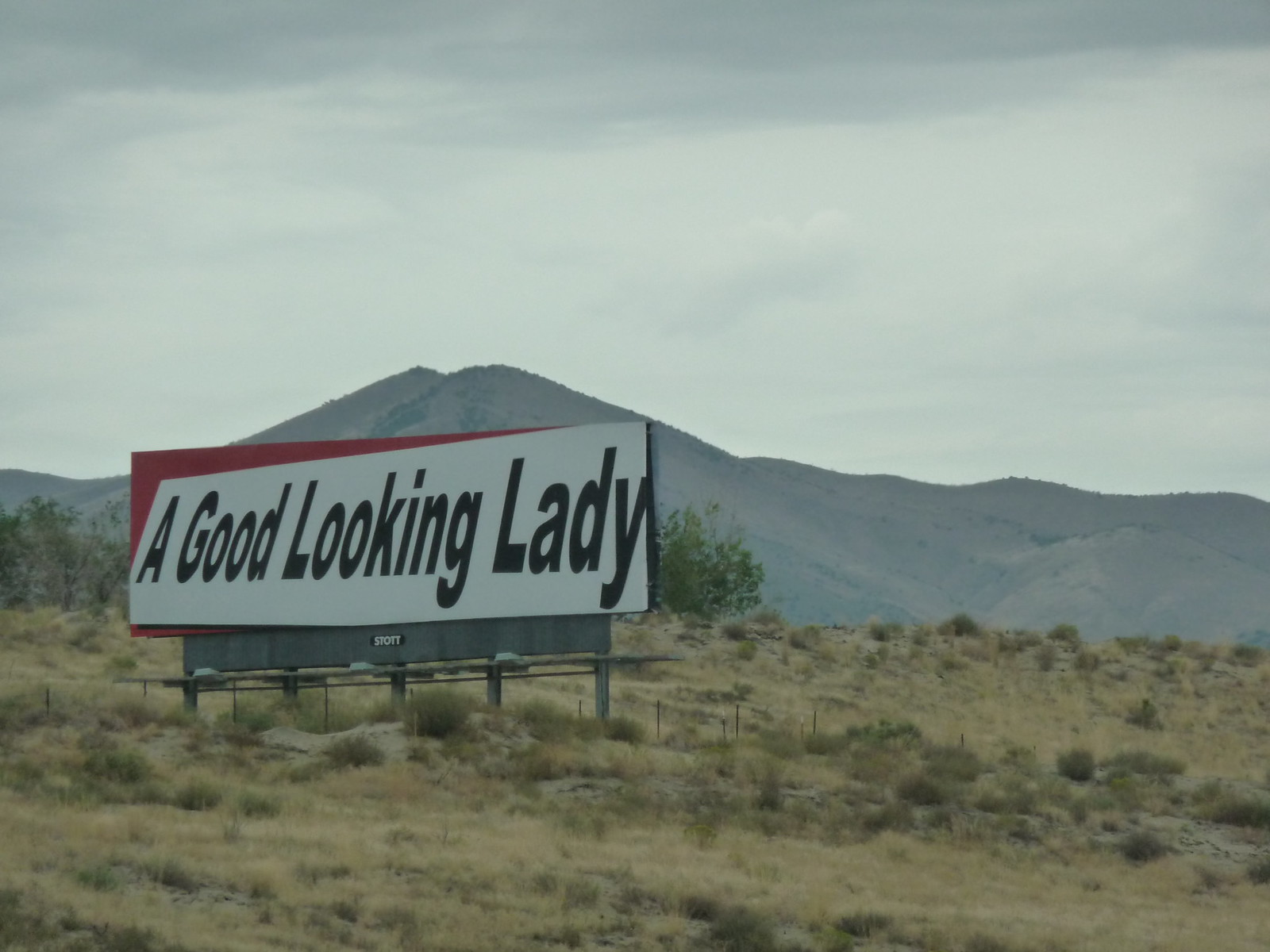A photograph captures the essence of the Southwestern United States, reminiscent of a scenic drive along historic Route 66. The setting could be in Wyoming, New Mexico, or perhaps where the desert meets the highways of Nevada or California. Dominating the scene is a large highway sign, prominently displaying the brand "STOTT, The Sign Company," against a white or light gray background. The sign features a vivid red trim extending from the top left corner across the top edge. Boldly inscribed on the sign are the words, "A Good Looking Lady," making a striking statement in the desolate landscape.

In the background, a low mountain range stretches along the horizon beneath an overcast sky. The foreground is characterized by sagebrush dotting a vast prairie, interspersed with fences that hint at the rugged, open terrain. The scene is framed by the barren beauty typical of this region, where expansive skies and remote wilderness converge. All elements combine to evoke a sense of nostalgia and solitude, symbolizing the timeless allure of America's open roads.